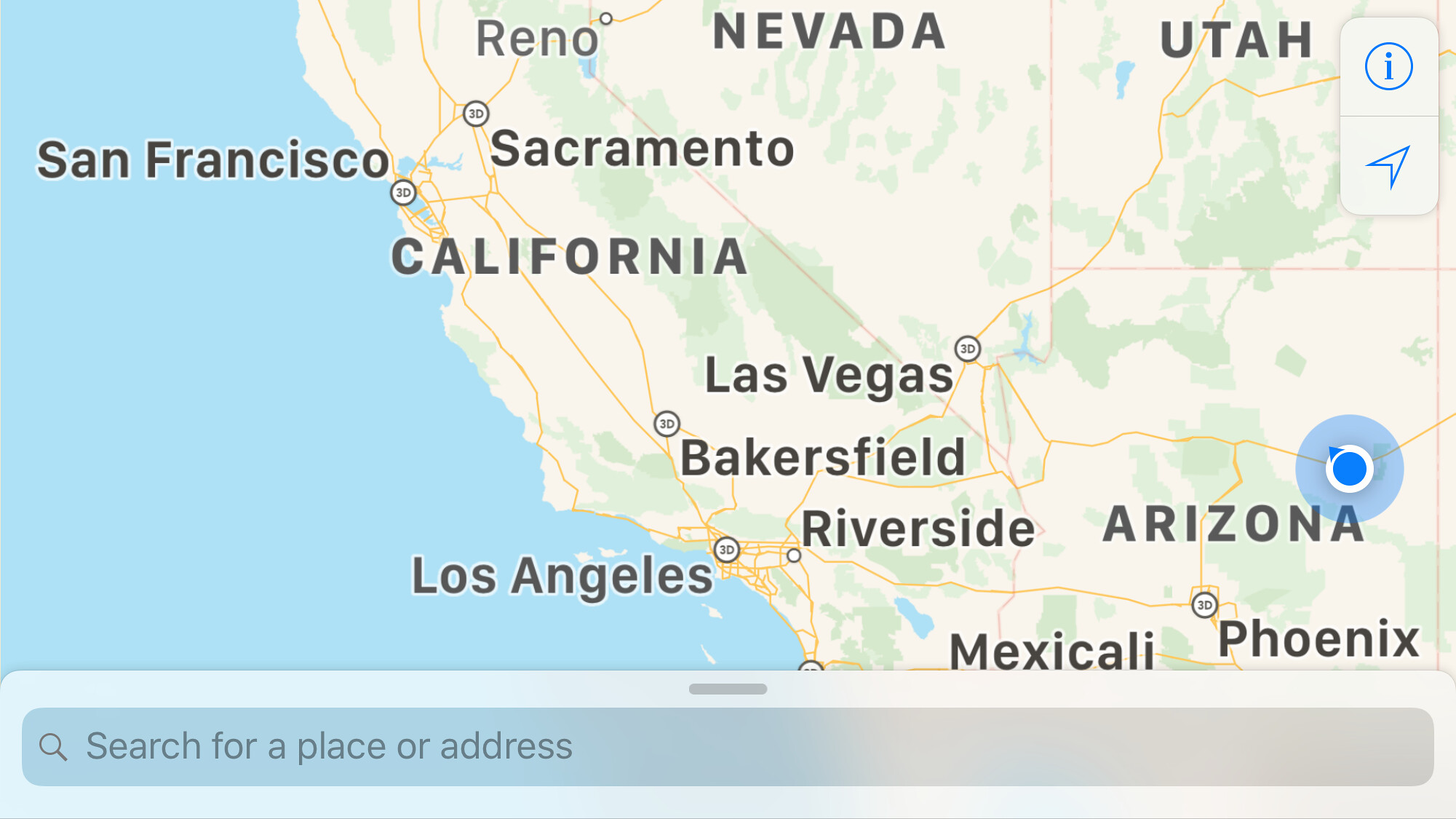This image is a screenshot of a digital map, likely taken from a Google or Apple Maps application. The screenshot prominently features a blue dot with an accompanying blue triangle, indicating the current location of the user in Arizona. The map spans a broad region, displaying parts of Arizona, Utah, Nevada, and California. While many Californian cities are labeled, the only city marked in Arizona is Phoenix. In Nevada, Reno is mentioned, and Utah remains unlabeled. To the left, the Pacific Ocean is visible, adding to the geographical context. At the bottom of the screenshot, a rectangular search bar is displayed, with text suggesting the user can "search for a place or address." This bar highlights the interactive nature of the map. The user appears to be near a major interstate, possibly Interstate 40, though the exact highway is not identified.